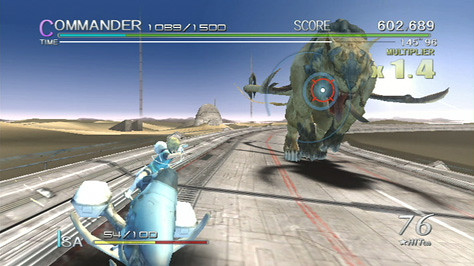The image appears to be a screenshot from a futuristic racing video game, displayed in a rectangular landscape format approximately two and a half times wider than it is tall. Dominating the scene is a road, specifically a two-lane highway with a distinctive red stripe running through the middle. This road extends from the foreground but then sharply curves to the right, disappearing from view towards the middle right of the image. On the left lane in the foreground, there is a blue motorcycle that the player seems to be riding. 

Taking up much of the right lane and heading towards the viewer is a menacing, large furry creature that resembles a woolly mammoth, suggesting it's about 20 feet tall within the game's context and appears to move menacingly towards the player. Above the scene, various game statistics are displayed in white text, including the word "Commander," accompanied by the figures "1099 / 1500," a score reading "602.689," and a multiplier "X 1.4" in yellow. 

The backdrop features a clear blue sky, contributing to the futuristic ambiance, and possibly hints at a space-themed setting. The overall graphics and layout suggest that it might be an older game, with a mix of cartoony and retro elements.